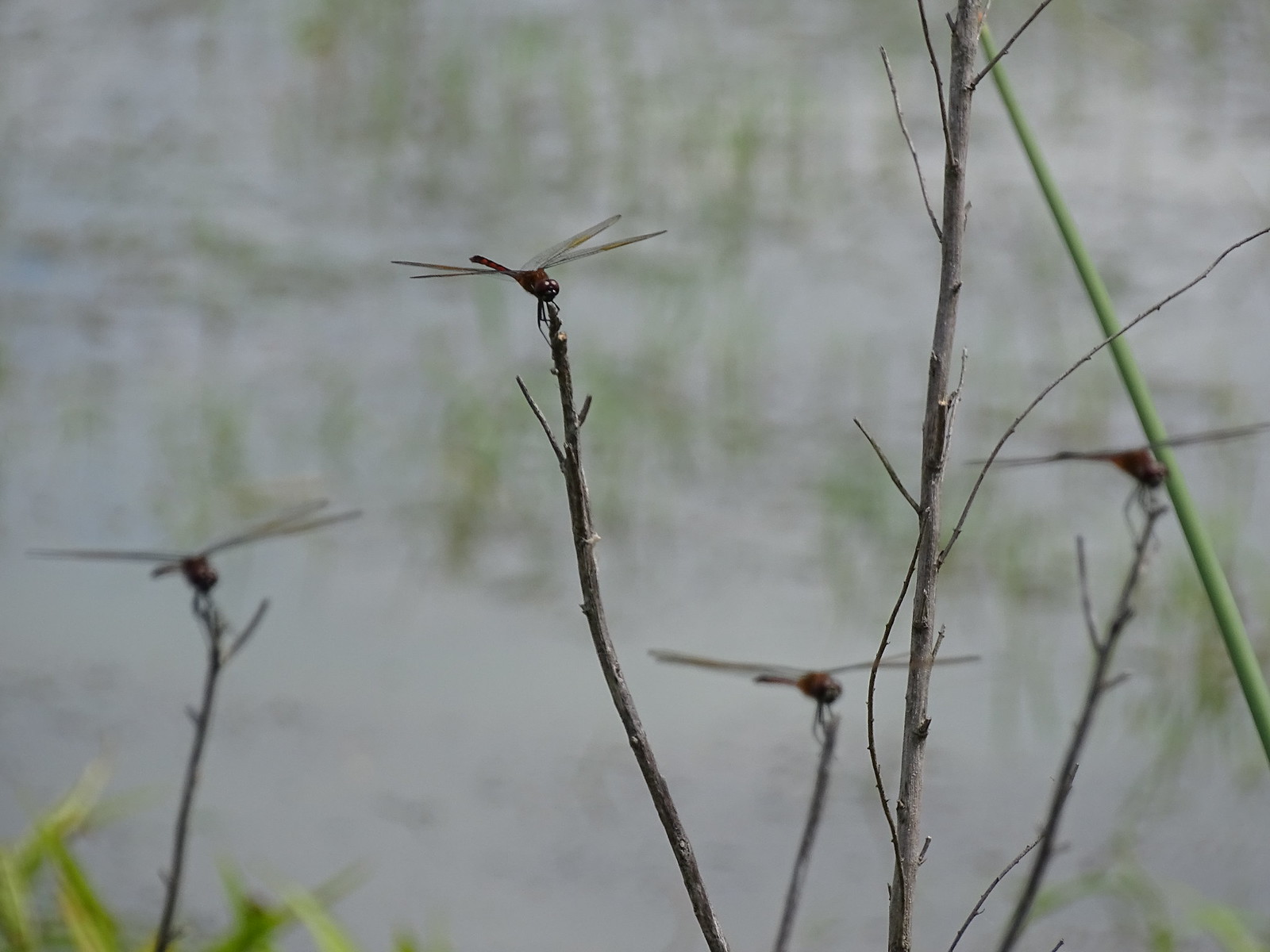The image depicts a detailed, up-close view of a swampy area, where the foreground elements are in sharp focus against a blurred background of green reeds and water. Prominently featured are five brown branches, emerging vertically from the ground, each adorned with a dragonfly. The dragonflies, totaling four and positioned towards the camera, display their distinctive clear wings fanned out on either side of their oval bodies with thin tails. One of the branches is particularly short, while another is slightly taller and ends in a V shape. Additionally, a slender green blade of grass extends diagonally from the bottom right corner of the photograph, adding to the composition. The muted colors of the blurred background contrast with the detailed textures and forms of the dragonflies and branches in the foreground, capturing the tranquil simplicity of this natural scene.